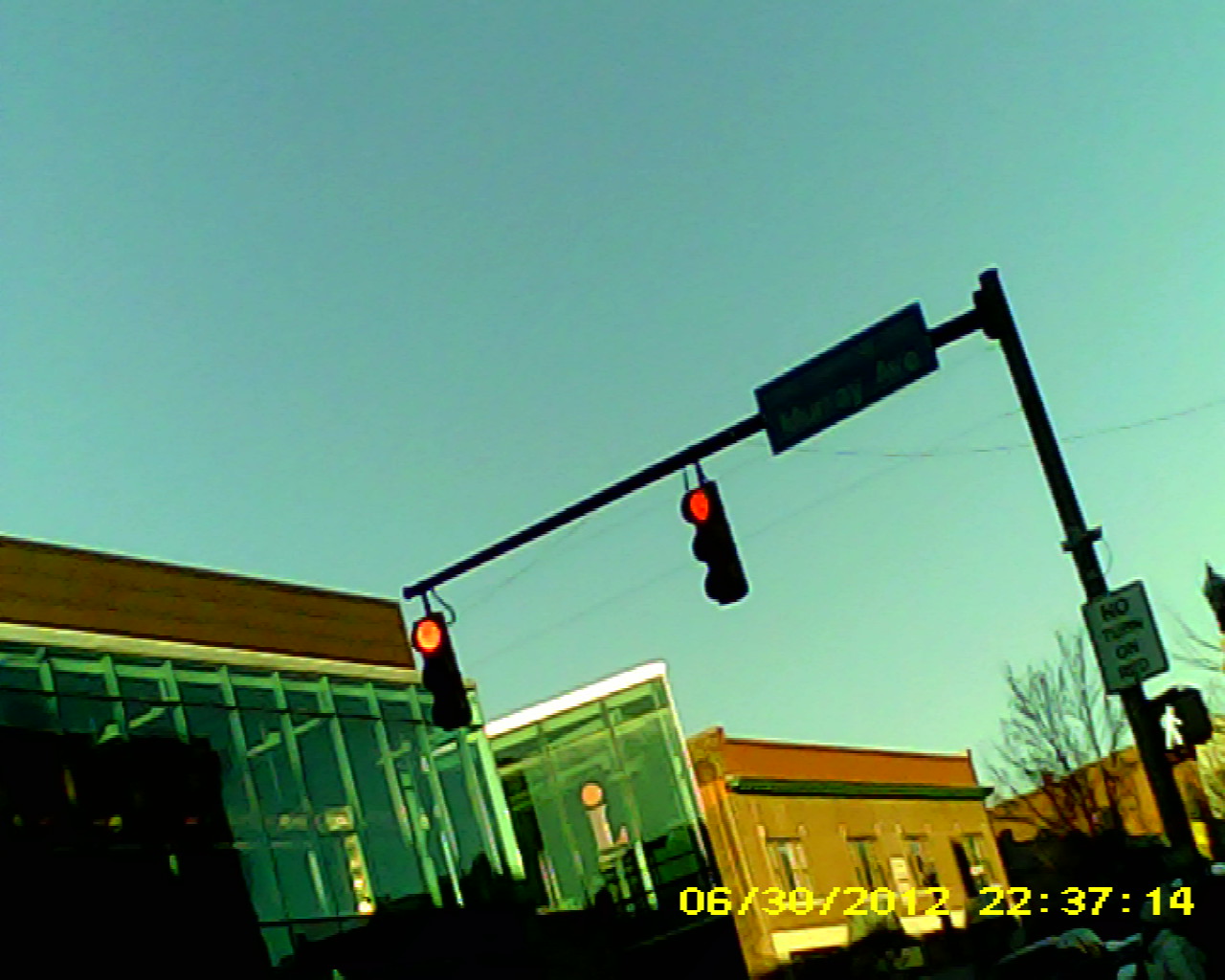The image features a pair of streetlights, each equipped with three circular lights, mounted on a tall pole. Both streetlights display illuminated red signals at the top. To the right of the streetlights is a black sign, possibly bearing a street name, though its content is illegible due to shadows. The pole itself, partially obscured by shadows, extends from the ground and bears a "No Turn on Red" sign. Below this sign, a smaller light indicates a crosswalk with an illuminated white pedestrian figure.

On the left side of the image stands a building with a brown trim and greenish windows, while to the right, another building, also brown with green trim, is visible. Adjacent to this second building is a skeletally bare tree. The lower section of the image includes indistinct black silhouettes, making it hard to discern specific details.

Above, the sky transitions from blue in the upper left corner to a lighter, whitish hue towards the bottom right. Scattered across the sky are power lines. Additionally, a timestamp watermark in yellow is located in the bottom right corner, denoting the date and time as 06/30/2012 and 22:37:14.